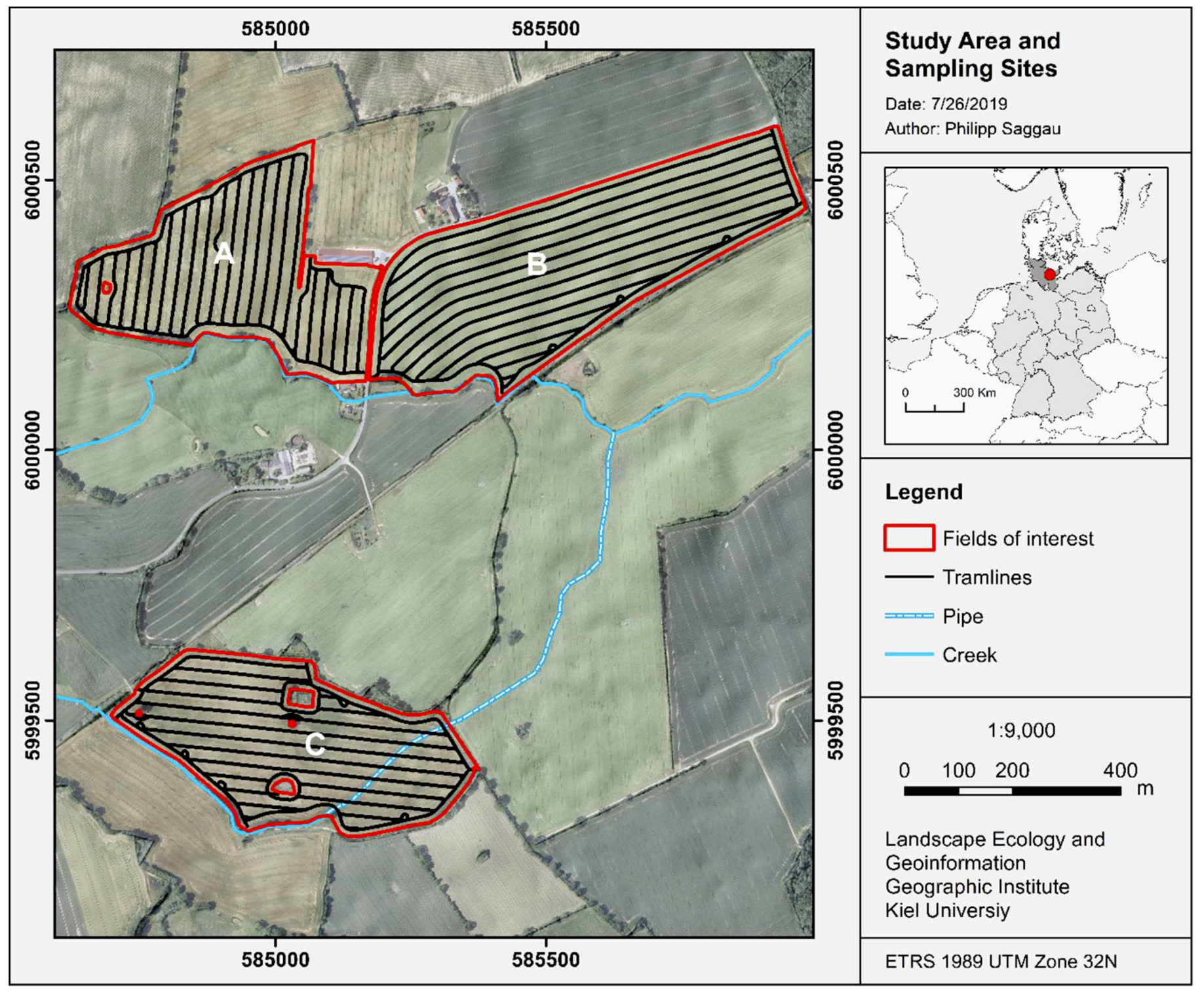This detailed geological chart and diagram map, authored by Philip Segal and dated July 26, 2019, focuses on a specific study area. Created by the Landscape Ecology and Geo-Information Geographic Institute at KL University, KIEL, the image primarily serves as a geographical survey tool. The map is color-coded to represent different features of the land, using red to denote the boundaries of fields of interest, black for tramlines, blue for creeks and thin, rectangular water pipes. The scale of the map is 1 to 9,000, with a distance of about an inch representing 400 meters. The layout is framed by a black border, with numerical coordinates along the edges; significant markings include coordinates like 585-000 and 585-500 towards the bottom center. Additionally, the top left coordinates extend from approximately 5,999,500 to 6,000,000. The map key includes labels for fields of interest, tramlines, pipes, and creeks, and does not feature any human images or real photographs. This detailed, aerial topography map is a high-resolution depiction used in the study of landscape ecology and geographic information systems.